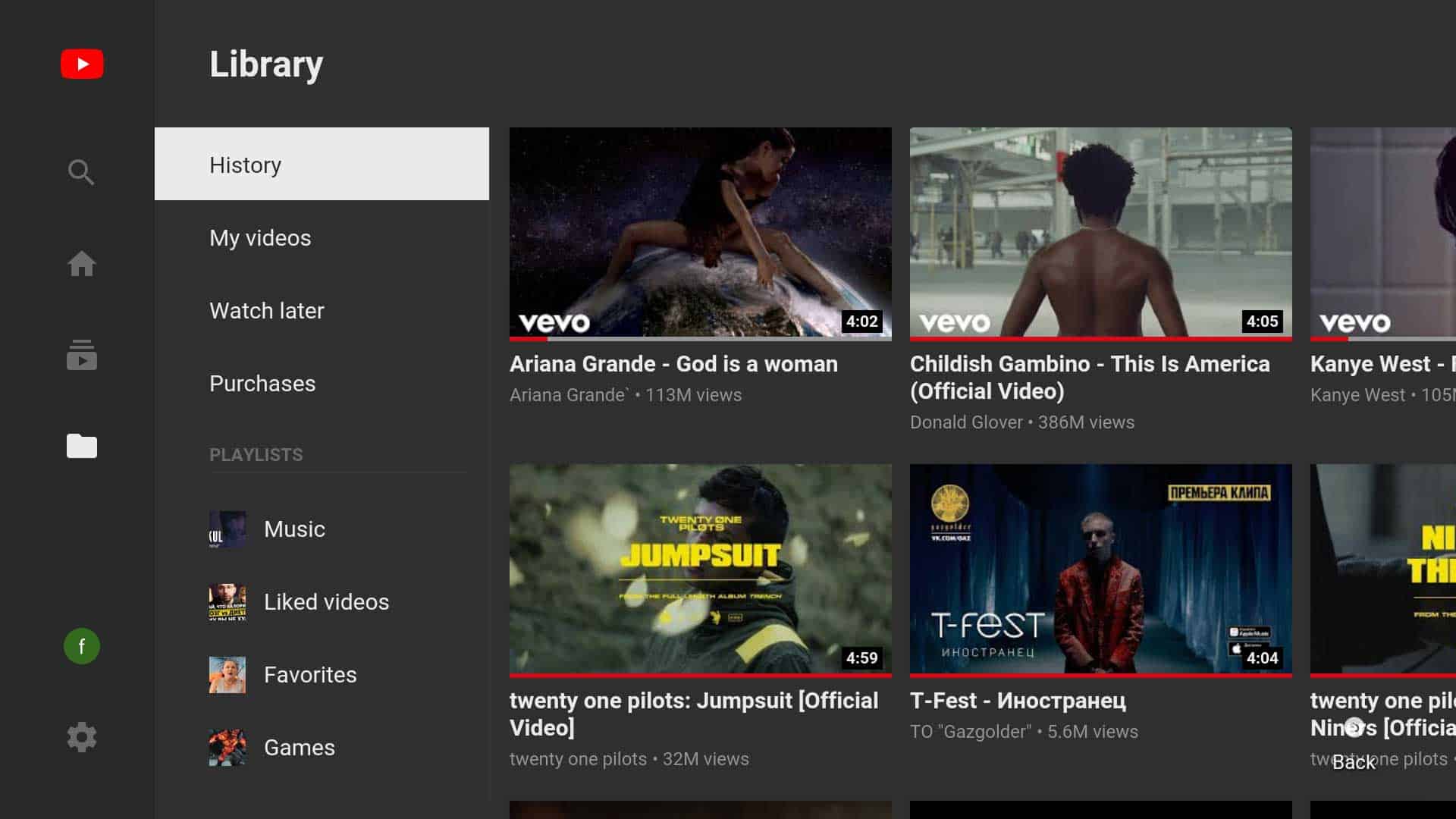This image is a screenshot of a YouTube video page, specifically displaying music videos. On the left side, a vertical row of several icons is visible. In the upper left-hand corner, a small red square featuring a white play triangle is present, indicating the YouTube logo. Below the logo, there are four icons, followed by a space, and then two more icons. Towards the bottom left corner, there's a gear icon. Adjacent to the gear icon is a menu column labeled 'Library' in white text on a dark gray background. The additional menu items listed are 'History,' enclosed in a white rectangle, 'My Videos,' 'Watch Later,' 'Purchases,' and 'Playlists.'

To the right of this menu column, the main content area features two rows of three thumbnail images each, representing different music videos. Each thumbnail includes the artist's name, the song title, and the view count below the thumbnail. In the lower right-hand corner of each thumbnail, the duration of the video is stated. Each thumbnail primarily showcases an image of the respective artist, offering a visual preview of the videos available to watch.